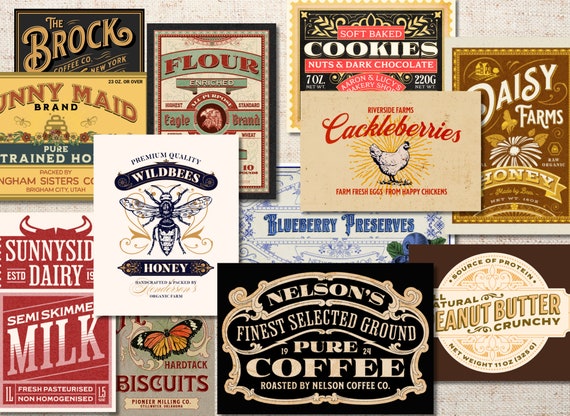The image is a collage of various overlapping product labels and logos, forming a vibrant, intricate canvas. The top left features the Brock Coffee CEO New York label in green with gold letters. Adjacent to it, there's "Flower Enriched Eagle Brand" with an eagle symbol and a "Soft Baked Cookies, Nuts and Dark Chocolate" label. "Daisy Farms Honey" is nearby, adorned with bees. Below, "Riverside Farms Cackleberries" displays a chicken, and a vibrant "All Natural Peanut Butter Crunchy" label peeks through. The center showcases "Nelson’s Finest Selected Ground Pure Coffee, roasted by Nelson Coffee Co.," within a tan insignia inside a black horizontal rectangle.

To the right, "Sunnyside Dairy Semi-Skimmed Milk" with bull horns above it stands partially hidden. Above it is "Wild Bees Honey," and to the side, a "Hard Tack Biscuits" label features a butterfly. Lower down, "Blueberry Preserves" is partially obscured, while at the bottom right, another honey label, "Sunny Made Brand Pure Strained Honey," is visible with a beehive depicted on it.

This dense assemblage of colorful, text-filled labels includes distinct references to various products like cookies, coffee, honey, milk, and peanut butter, making it a richly detailed, busy mosaic of commercial art.